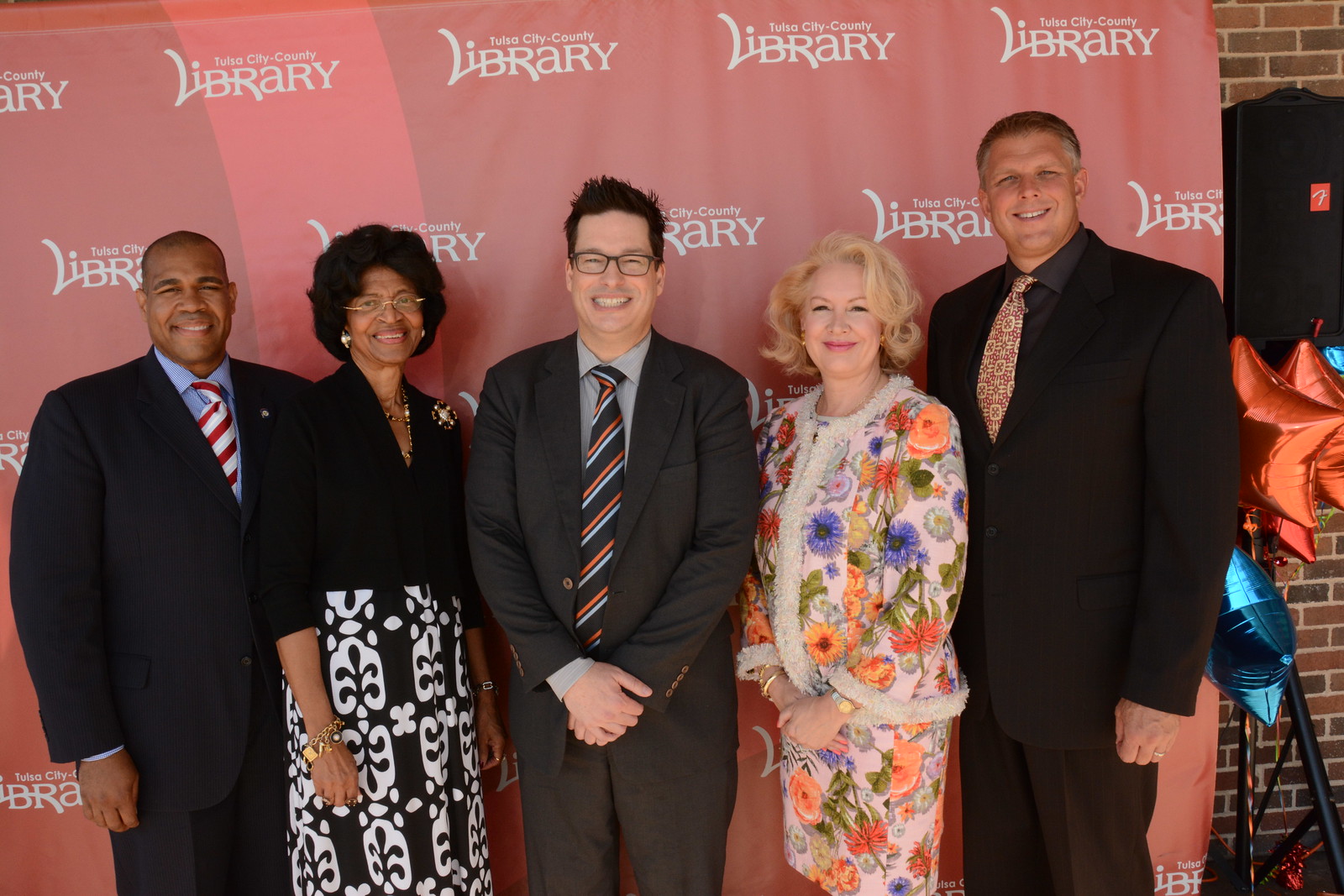This image features five individuals standing in front of a salmon-colored backdrop adorned with the repeating text "Tulsa City County Library" in a distinctive white font where the 'L' in 'Library' stretches across the 'IBR', creating a unique design. From left to right, the individuals are:

1. An older African American man, who is bald and smiling, donned in a black suit jacket, blue shirt, and an American flag tie featuring red and white stripes.
2. Next to him stands an older African American woman with glasses and voluminous black hair. She wears a black sweater over a long black and white dress with fleur-de-lis patterns.
3. The central figure is a Caucasian man with spiky black hair, black glasses, and a bright smile. He is dressed in a dark gray suit, a tan shirt, and a tie with red, white, and blue stripes.
4. To his left is a blonde Caucasian woman, smiling, with a floral print ensemble that includes a skirt and a top detailed with orange and blue flowers.
5. The tallest person in the group is another Caucasian man, wearing a black suit, black shirt, and a peach and white patterned tie. 

The background also features assorted elements such as red and blue star-shaped helium balloons, some positioned near a black speaker on a pole, indicating an outdoor setting with a hint of celebration or event ambiance.